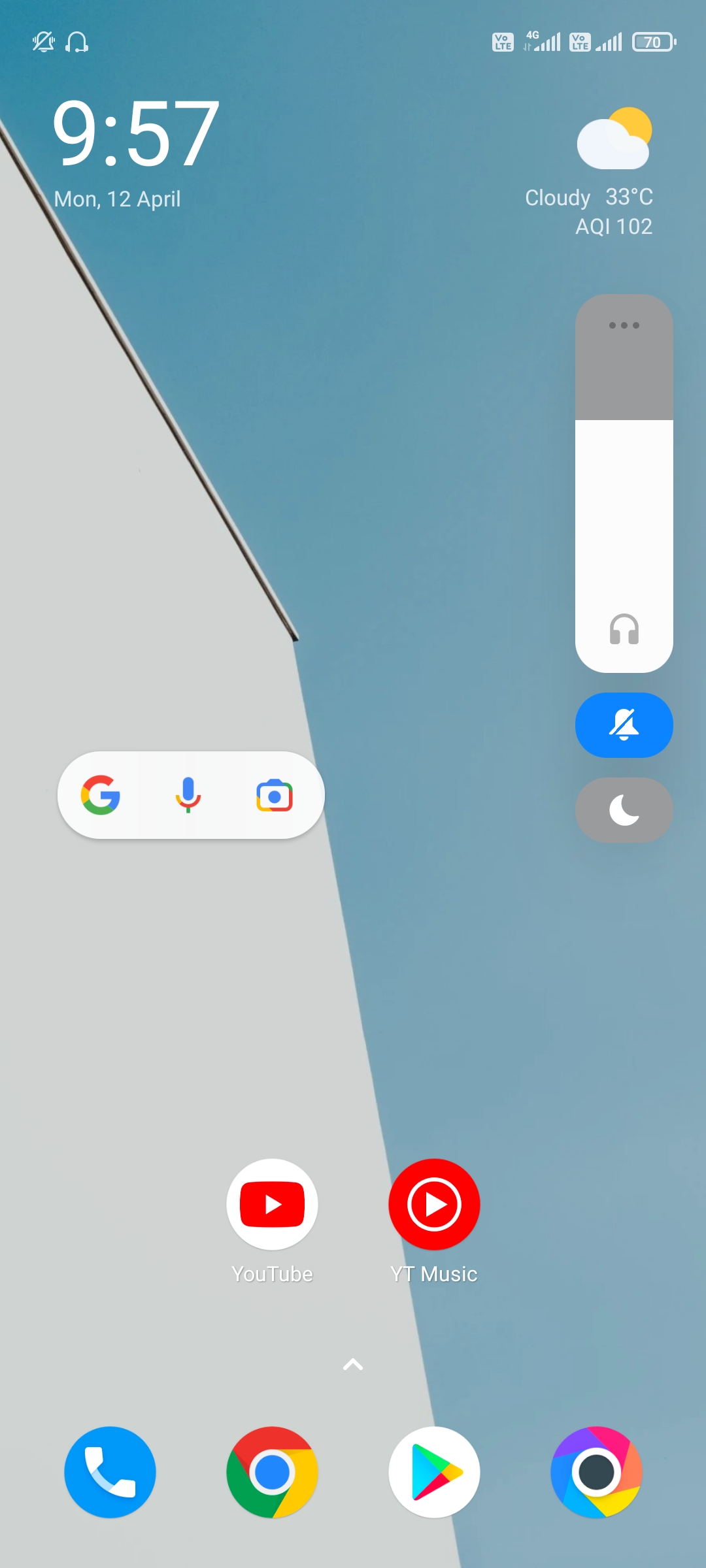A smartphone display shows the home screen featuring the date and time "Monday, 12th April, 9:57." The weather widget indicates cloudy conditions with a temperature of 33 degrees Celsius, accompanied by an icon of a sun partially obscured by clouds. The background photo on the screen depicts a gray building against a bright, clear blue sky. 

To the right, an earphone icon suggests the volume is set at around 75-80% for headphone output. The center of the screen displays several application icons: a red "G" for Gmail, a speakerphone icon, an unidentified logo that might represent Google Photos or a camera, and the YouTube icon, which features a white triangle within a red rectangle. Adjacent to these is the VT Music app icon represented by a red circle containing a white triangle within another white circle.

At the bottom of the screen, there are four symbols: a blue phone icon, the Google Chrome icon, and two other indistinct symbols.